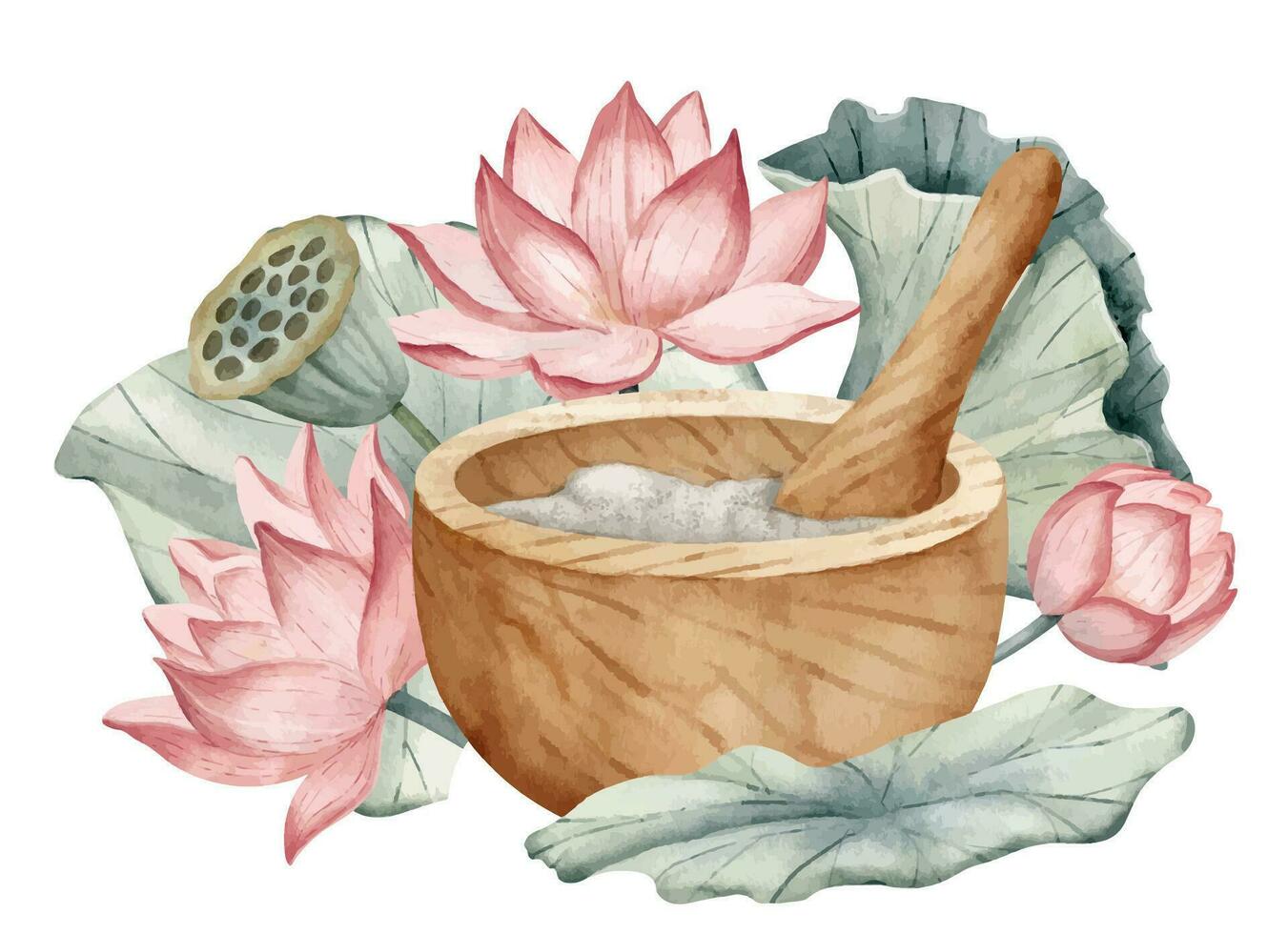This detailed painting features a wooden, cylindrical mixing bowl in the foreground, containing a white powdery substance that resembles flour. A wooden spoon or stirring stick protrudes from the bowl. Surrounding the bowl are beautifully vibrant green leaves and pink lily pad flowers, with their petals mostly open in full bloom, though one on the right remains in a bud-like state. Among the foliage on the top left of the bowl is a distinctive plant resembling a honeycomb, with a green bulb that appears to be cut in half, showing holes within. The colors in the painting are a harmonious blend of pinks, rose, turquoise, and grays, adding a serene yet vibrant touch to the scene.